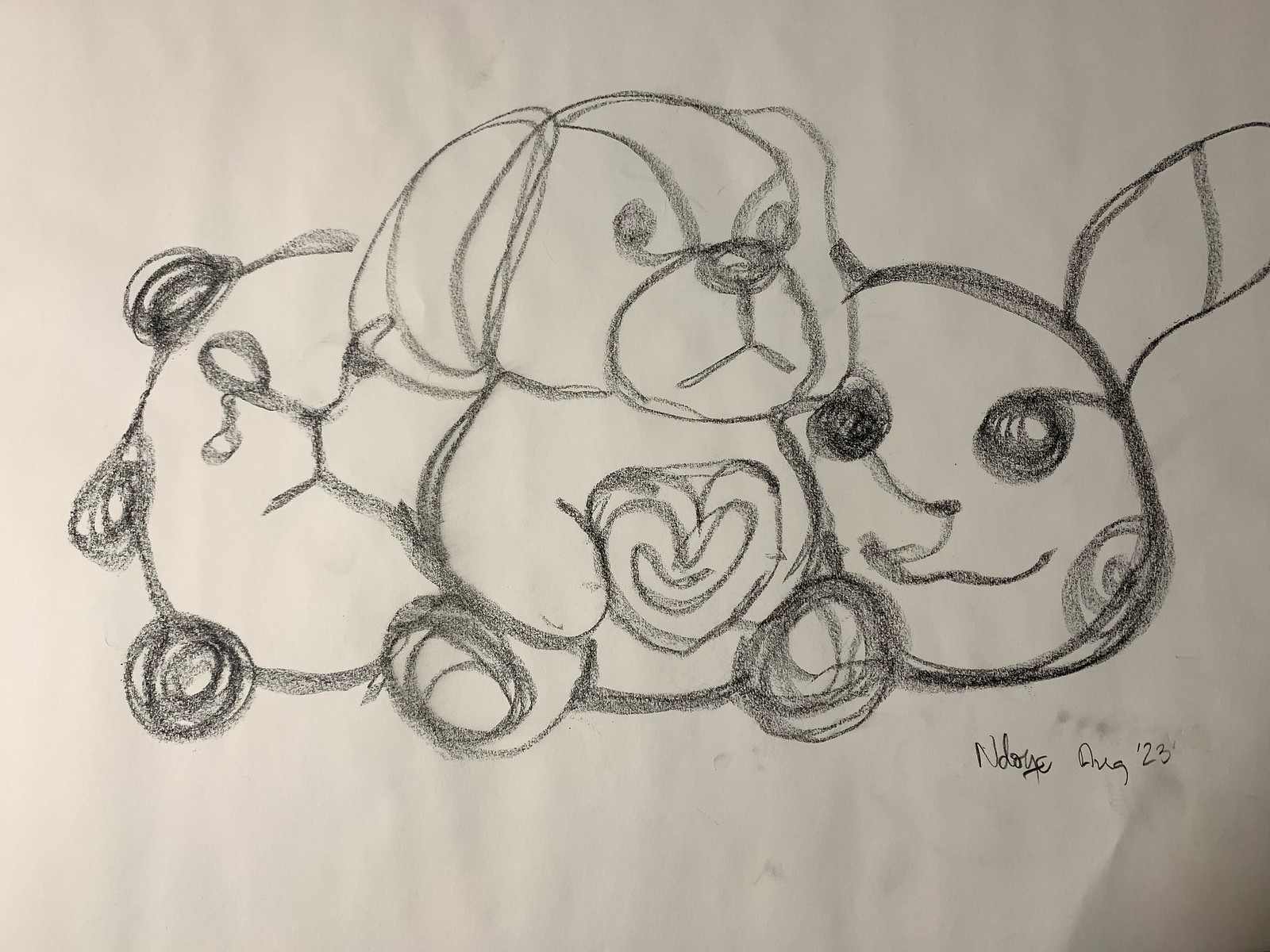The photograph captures a child's playful drawing on a white sheet of paper, rendered in black crayon or charcoal that imparts a sketch-like quality. Central to the drawing is an expressive dog with floppy ears, a circular body, large eyes, a prominent snout, and a heart on its tummy. On the right side of the dog is another animal, likely a rabbit, characterized by large round eyes, prominent long ears, and distinctive spiral cheeks. On the left side of the dog is a figure that appears to be a crying panda bear, distinguished by its round ears, circular body, and paws. The drawing is signed "Ndoye" in the bottom right corner and dated August 2023.